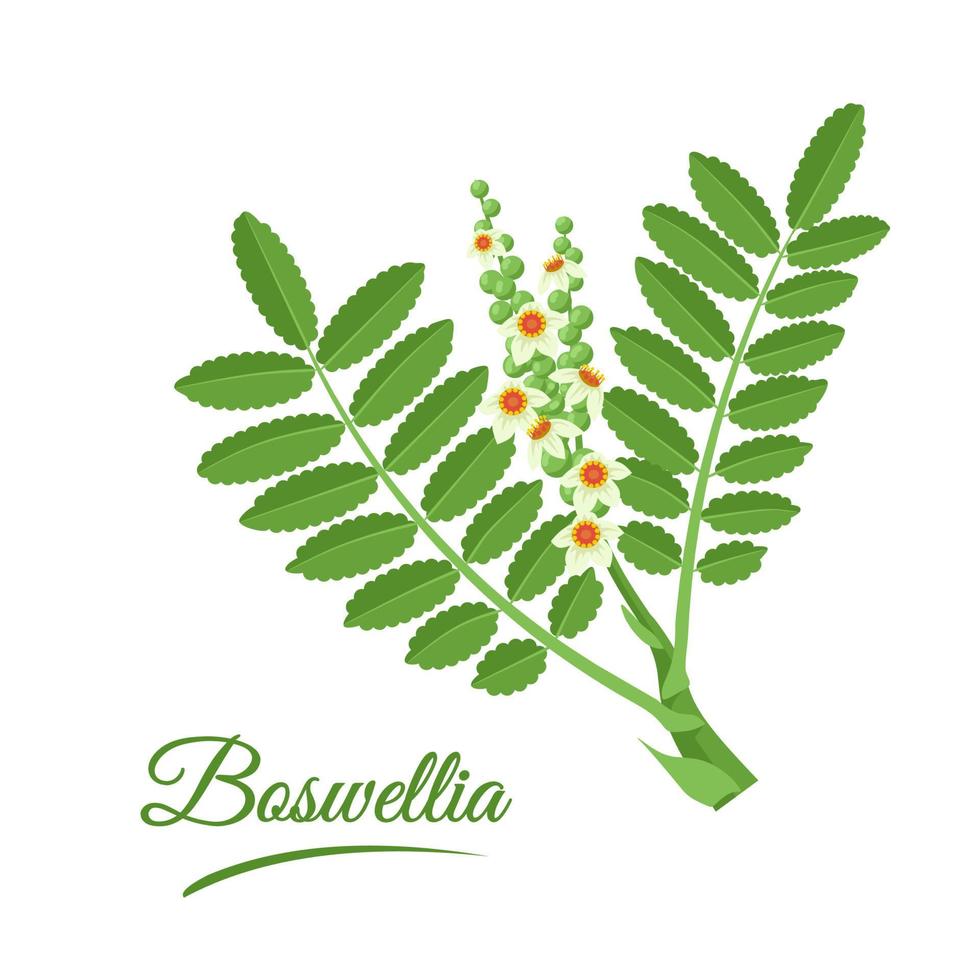The image showcases a detailed graphic depiction of the Boswellia plant, prominently labeled in cursive "Boswellia" in green in the bottom left corner with an underline. The plant features green, serrated, bay-like leaves that grow in pairs along the vine, alternating horizontally with the occasional vertical branch. The leaves are bordered with small, bead-like structures. Among the foliage are numerous budding flowers with yellow petals and sunburst orange centers, some with tiny yellow dots at their cores. The branches, stems, and leaves are depicted in a vibrant green, while the flowering parts stand out with their vivid yellow and orange hues. The overall composition suggests a mix of natural illustration and artistic representation, likely intended for educational or promotional purposes.